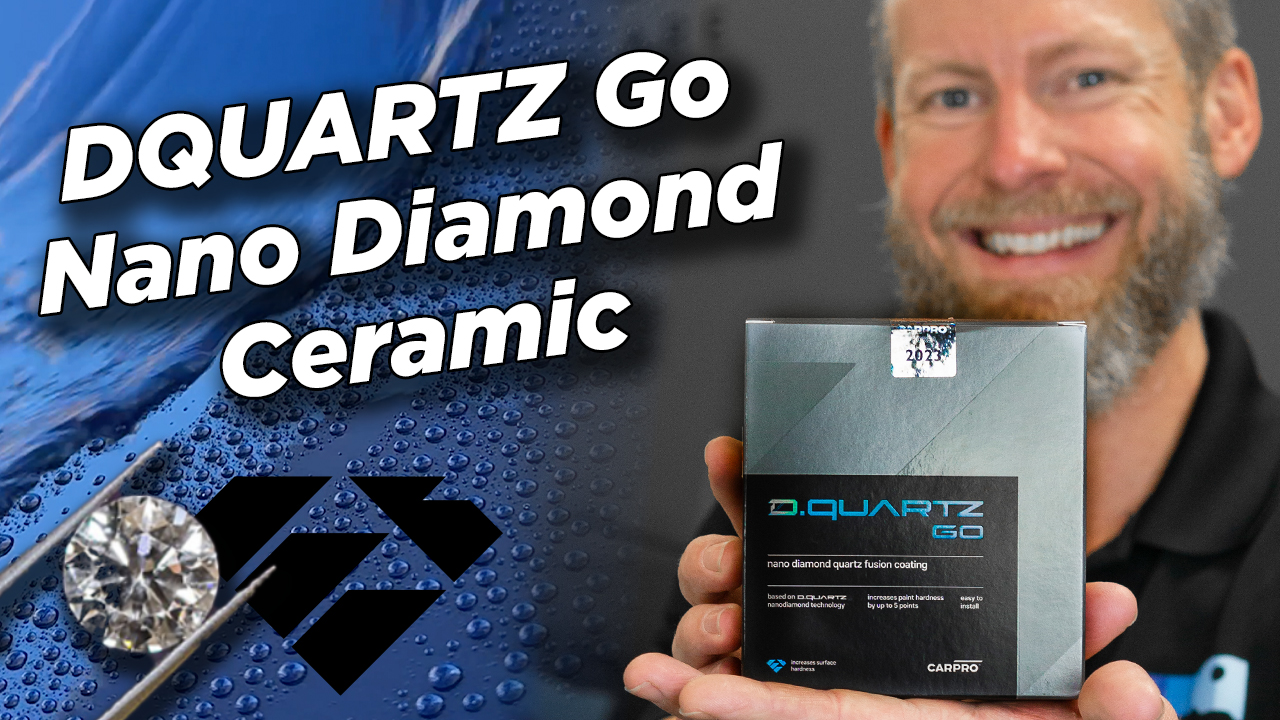This photographic image appears to be an advertisement for a product called "D Quartz GO." The central figure is a smiling white man with a gray beard and mustache, looking directly at the camera while holding a box. The box features prominent text that reads, "D Quartz Gold, Nano Diamond Quartz Fusion Coating," and includes further details about the product’s benefits, such as increased point and surface hardness due to its Nano Diamond technology.

The top left corner of the image features the brand name "D Quartz Gold" in bold white text, alongside the phrase "Nano Diamond Ceramic," indicating the nature of the product. Below this, a diamond, held delicately by a pair of tweezers, is depicted against a backdrop of a blue, possibly automotive surface adorned with water droplets. The box the man is holding complements this visual theme with teal and blue tones, reiterating "D Quartz GO" and related product information.

The bottom right corner of the box displays the brand "Capro 2023," while additional small text, likely instructions or further specifications, is noted but too small to be clearly read. Overall, this image combines a visually engaging layout with detailed textual information to effectively promote the D Quartz Gold Nano Diamond Quartz Fusion Coating product.